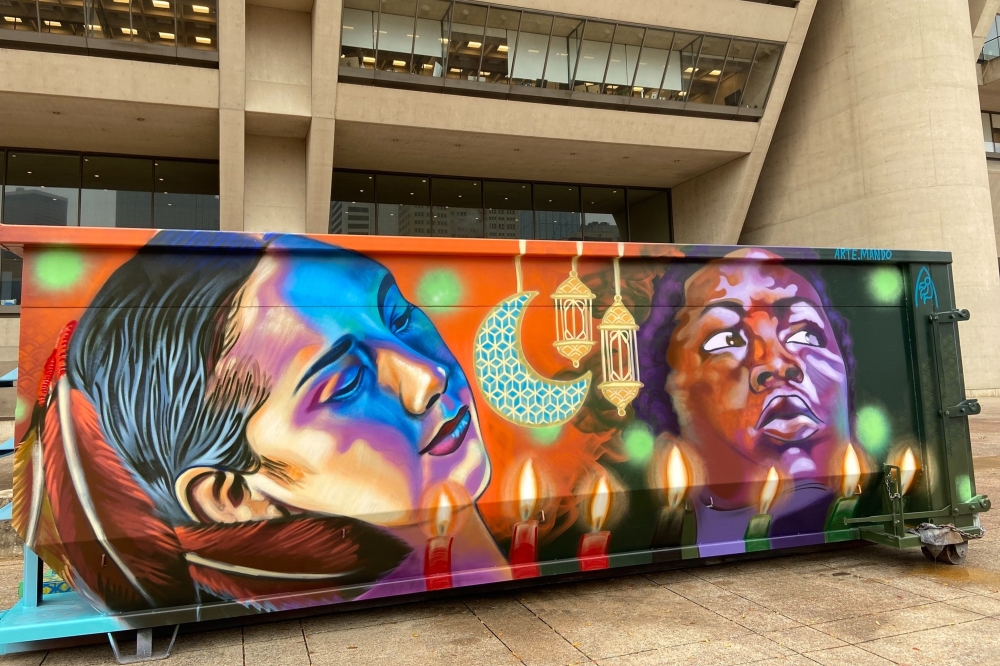A vibrant mural adorns a large, clean green dumpster situated in front of a modern-looking office building with glass windows, possibly indicating an urban setting. The mural features two women, the one on the left possibly Native American or Hispanic, identifiable by the red feathers in her hair. The woman on the right appears to be either African American or Afro-Latina, standing beside a crescent moon adorned with a mosaic pattern and two ornate, Moroccan-style gold lanterns. At the bottom of the mural are seven lit candles, arranged in what seems to be a Kwanzaa setup, with three red candles, two green candles, and a single black candle. The dumpster’s original green color peeks through parts of the mural, and the name of the artist, "Arte Manudo," is signed on the artwork. The backdrop of the brown office building adds a contrasting, modern touch to the captivating, colorful image painted on the dumpster.